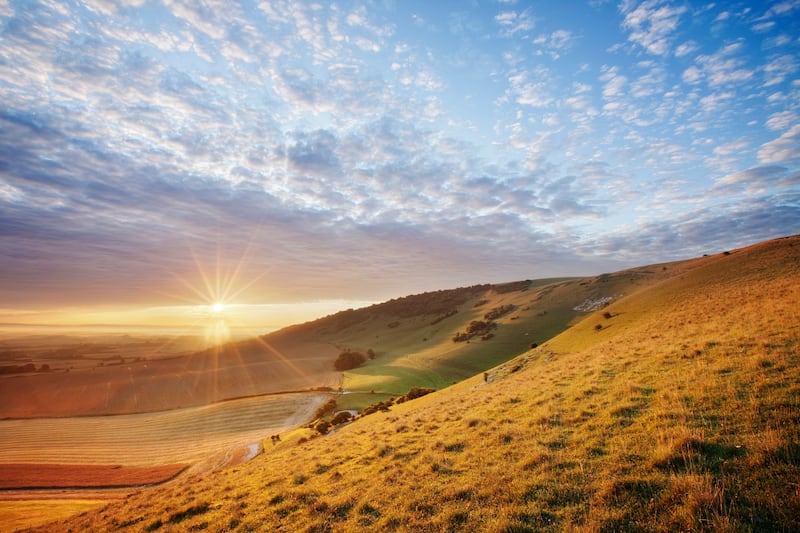The image depicts a vast, picturesque landscape during the daytime, characterized by a blue sky adorned with a mix of feathery, white clouds and some grayish ones in the distance. The sun is visible, positioned toward the horizon, casting an orangish-yellow light that suffuses the clouds, making them appear both gray above and orange below. The scene includes a large, grassy hill dominating the right side of the image, sloping down gently into a valley on the left. The grass across the hill and valley ranges in color from yellow-green to brown. Interspersed throughout the landscape are patches of trees and bushes, with some clusters growing more densely in certain areas. In the lower part of the scene, there are neatly organized rows resembling a crop field, indicating agricultural activity. The entire area appears untouched by human presence, as there are no visible signs of houses, people, or animals, lending a serene and unspoiled quality to the image. Ray of sunlight burst through the clouds, highlighting the tranquility and natural beauty of this rural setting.